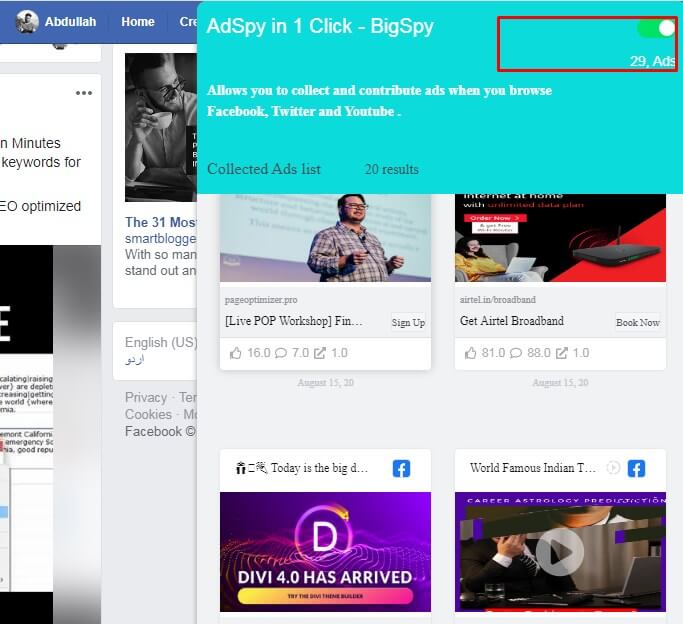The image shows a pop-up ad overlaying a Facebook interface, confirming it is from a period before Facebook's rebrand to Meta. The pop-up ad occupies much of the screen, with Facebook's familiar blue banner at the top displaying the user's name, Abdullah. Below, the screen reveals a teal banner with the title, "Ad Spy in one click, Big Spy." This banner informs users that the application allows the collection and contribution of ads while browsing Facebook, Twitter, and YouTube. The teal banner also includes a red box indicating that 29 ads have been collected, followed by a "Collected ads list" with 20 results.

The pop-up features four smaller images, all emblazoned with the Facebook logo. Part of these images showcases recently captured ads, including titles such as "Live Pop Workshop," "Get," "Airtel Broadband," "Divi 4.0 has arrived," and "World Famous Indian something." This suggests that the application serves as a tool for users, likely developers or advertisers, to track and analyze advertisements across various social media platforms.